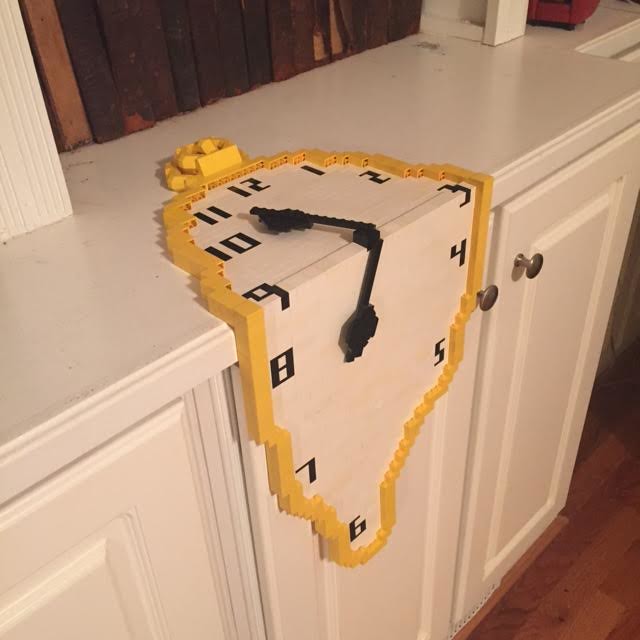This photograph features an intricately constructed Lego clock that appears to be melting, reminiscent of Salvador Dalí's surrealist artwork. The clock's frame is rimmed in gold or yellow and drapes fluidly over the edge of a white piece of furniture, which resembles a cabinet or an island with a dark iron or silver drawer pull. The face of the clock is white, adorned with black numbers and hands, each tipped with arrows. Notably, the clock’s numbers start at 12 and circle around, with the six uniquely drooping to the middle bottom of the cabinet, while the big hand points to 11 and the small hand to seven. The setting includes medium brown hardwood floors and an indeterminate dark blue window covering, possibly blinds or curtains, in the background.